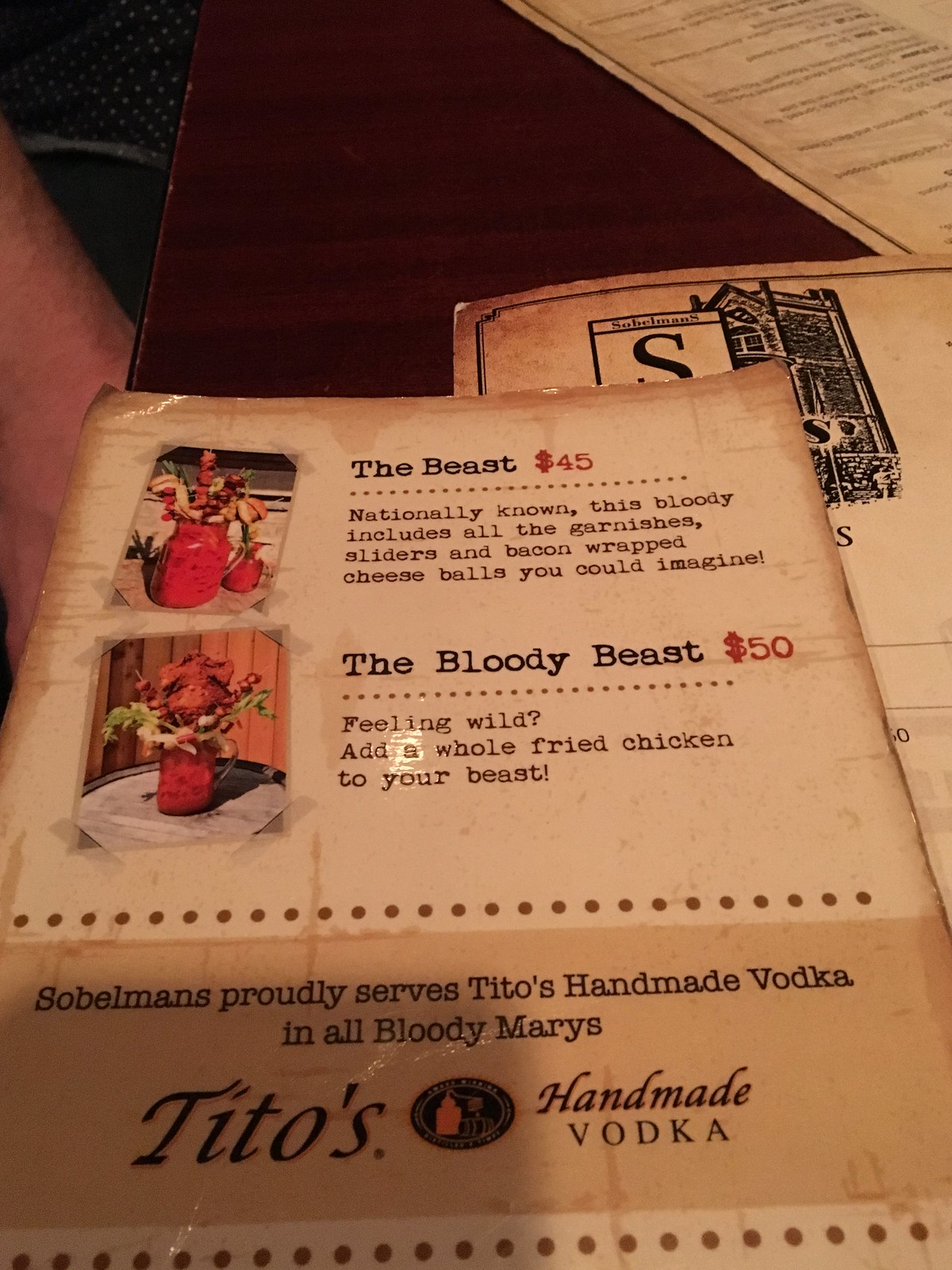The image showcases the back of a menu placed on a brown wooden table. The menu itself is situated with its upper right corner approximately two inches from the top of the frame and two and a half inches on the left. It spans diagonally past the middle of the image, creating a distinct presence on the scene. The menu is divided into different color zones: the upper portion is light brown, framed by a dark brown border on the top and sides, while the bottom third transitions into an even darker brown hue.

Prominently displayed on the upper left of the menu is a vibrant red drink garnished with assorted fruits. This drink, named "The Beast," is priced at $45. Adjacent to it, detailed in black lettering, is a description of the beverage. Below this, on the left side, sits another red drink with additional trimmings, named "The Bloody Beast," priced at $50. Beneath this, a text describes the inclusion of Tito's Vodka.

In the background, partially visible, are fragments of other menus. One, just beyond the top right corner of the primary menu, features a glimpse of a building. Another menu peeks from the right side and angles diagonally across the middle left portion. Adding to the scene, at the left center edge of the image, a forearm subtly extends under the table, contributing to the composition’s depth and human element.